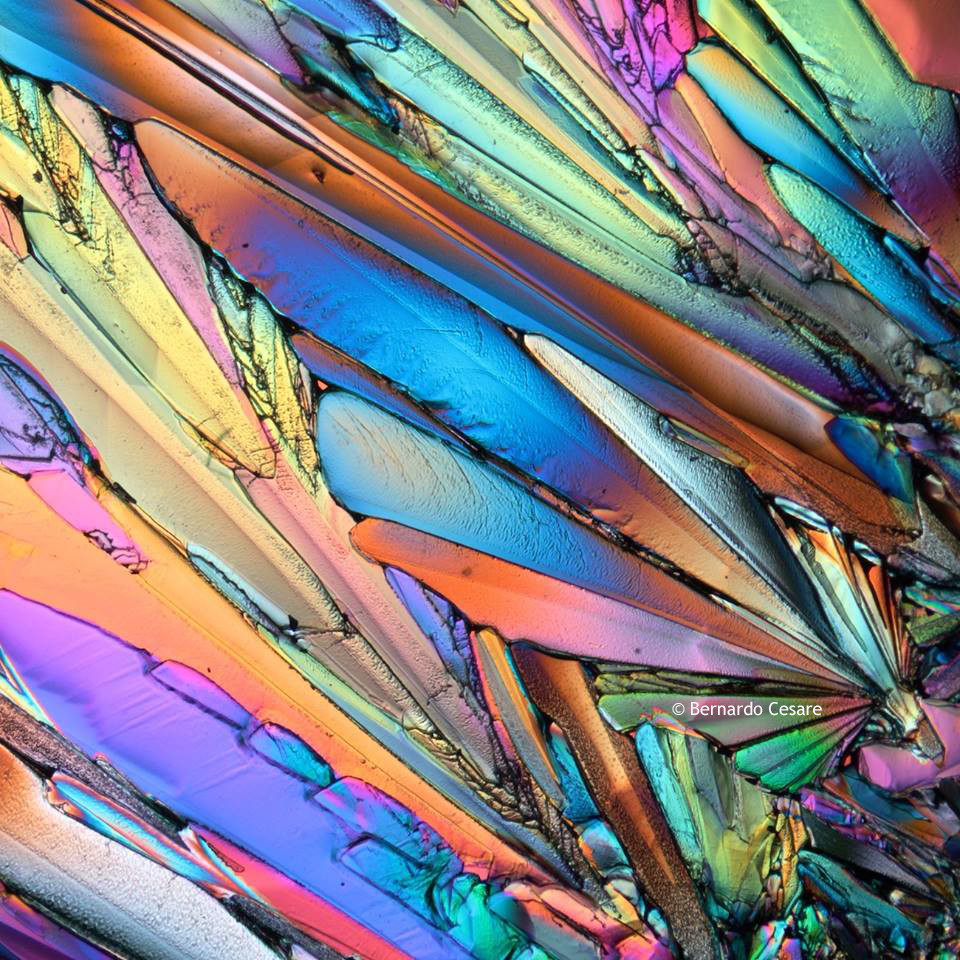This large square image showcases a vibrant and intricate array of colorful, iridescent objects that resemble long, narrow feathers with blunt, serrated edges. The feather-like shapes fan out in various directions, predominantly from the bottom right to the top left, and are adorned in a dazzling spectrum of colors including blue, orange, yellow, green, and purple. In addition to the feather forms, there are more geometric, fractal-like shapes superimposed over them, adding depth and complexity to the composition. The overall appearance suggests a blend of crystalline structures or perhaps the detailed pattern of a magnified insect wing, reflecting light in a highly colorful and reflective manner. In the lower right corner of the image, there is a copyright notice with the name "C. Bernardo Cesare," identifying the photographer.